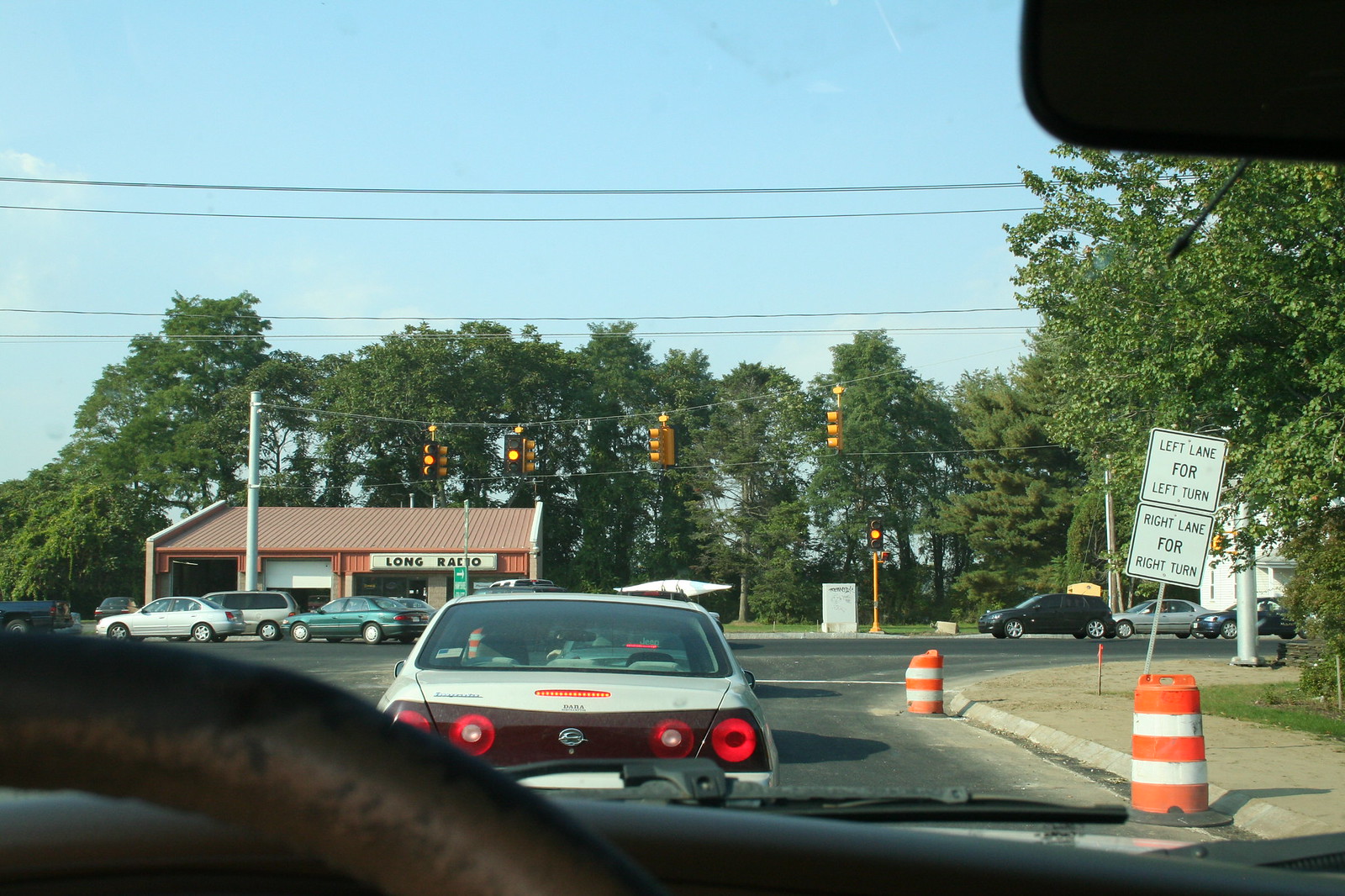This photograph, taken from the driver's seat inside a car through the windshield, captures a bustling street scene under a clear blue sky. The view is framed by the steering wheel and includes part of the dashboard and rearview mirror. Directly ahead, a white Chevy Impala, its red brake lights visible, waits at a yellow light of an intersection. The traffic is directed by stoplights supported by white poles, some of which show a yellow signal. 

To the right, construction barrels line the curb, guiding the traffic flow. The road splits into two directions marked by signs indicating "left lane for left turns" and "right lane for right turns". To the left, a sidewalk runs parallel to the street, featuring another sign with lane instructions. 

In front of the stopped cars, a small building bearing the name "Long Radio" stands, its garage bays partially open. Various vehicles in cross traffic display colors like white, green, black, and gray. The backdrop is dotted with leafy green trees, suggesting warm weather, while power lines crisscross the sky, adding to the urban landscape.